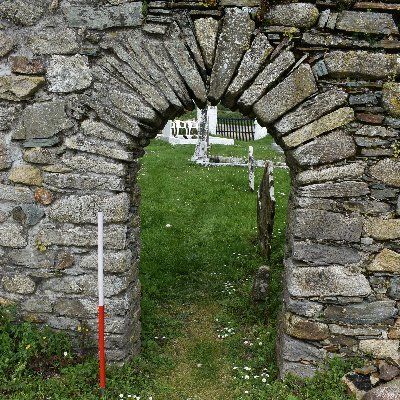The image depicts a large stone wall with an archway at its center, built from a variety of gray and white stones. This archway, resembling a door but without an actual door, offers a clear view through to the other side. Inside the archway, there is lush green grass and a black wrought iron fence, distinguished by white pillars. The photo is taken outdoors during the daytime, as indicated by the natural daylight illuminating the scene. To the left front of the stone wall, there is a prominent pole that is red on the bottom and white on the top. The surrounding area is covered in vivid green foliage, including small white flowers scattered across the grass, which contributes to the overall serene and historic atmosphere, possibly suggesting the location is a park, heritage site, or cemetery. The entire scene is framed within a square format, capturing the detailed textures of the stone wall and the verdant landscape beyond it.